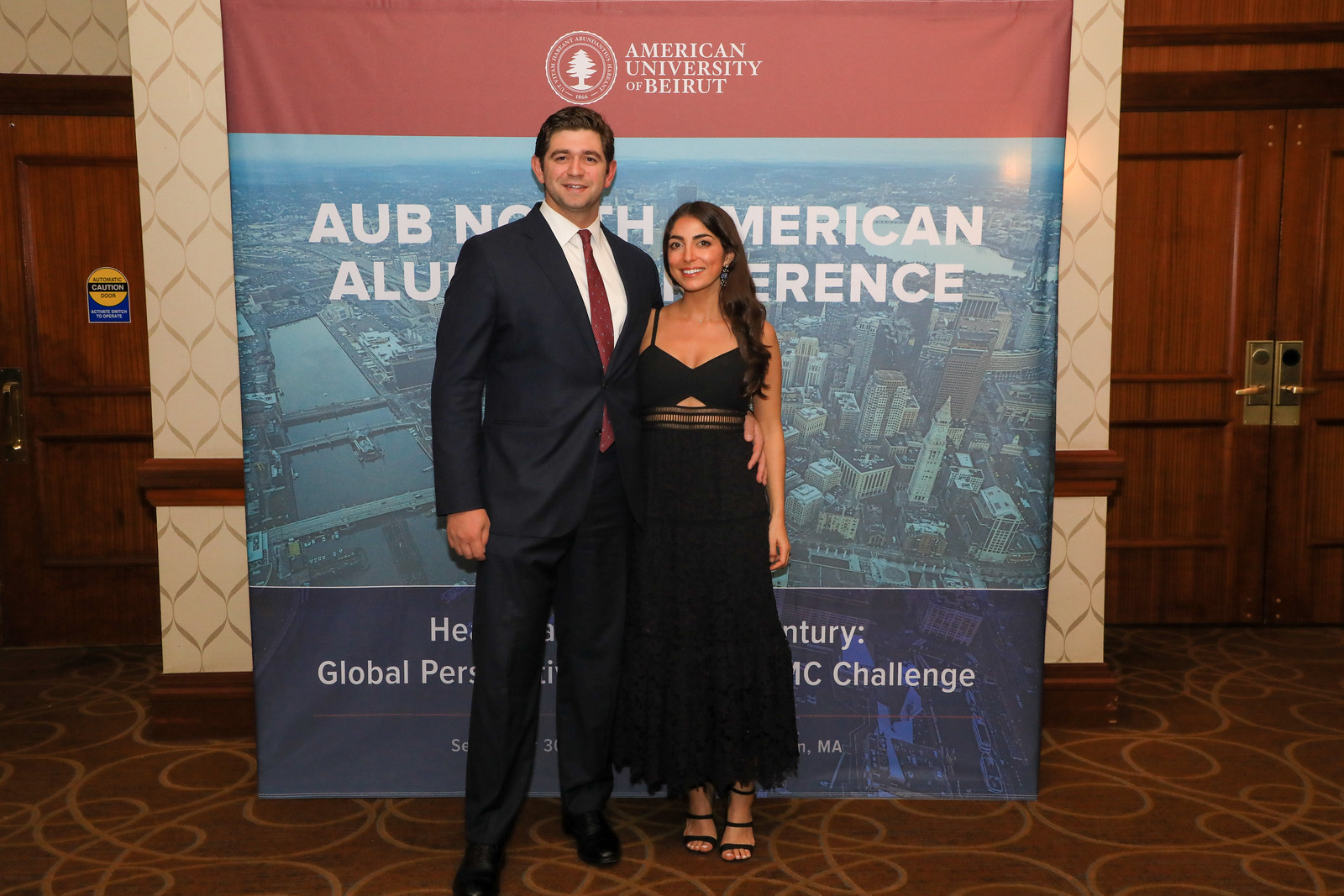A sharply dressed man and woman are standing and smiling for the camera at a formal event. The man, sporting a navy blue suit with a white button-up shirt and red tie, has short brown hair and dark eyes, and he has his arm around the woman beside him. She has long, dark brown hair and is elegantly dressed in a long black dress with a cutout detail and black sandals. They are posing in front of a banner with a red top section that reads "American University of Beirut," accompanied by the university seal. The middle part of the banner, blue with an aerial view of a city likely to be Beirut, partially reveals the phrase "AUB North American Alumni Conference" as it's partly obscured by the couple. The background includes a wall with a zigzag design and a dark brown carpet with light squiggle patterns, flanked by wooden doors on both sides of the pair.